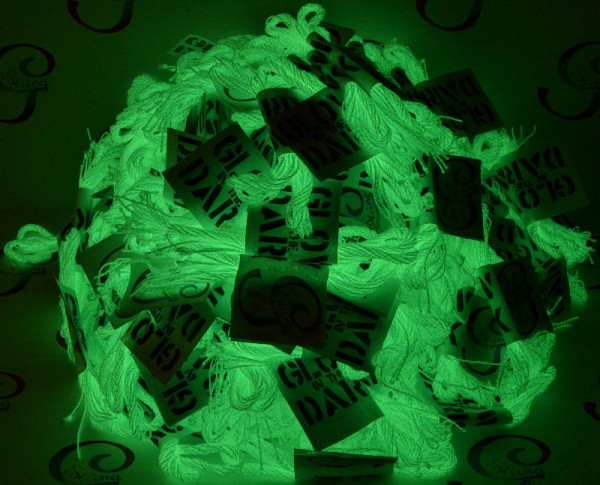The image features a striking green design set against a dark backdrop of black and deep green hues. The central element is a dynamic, fluorescent green pattern, comprising intricate, swirling shapes that evoke the impression of tangled forms, reminiscent of an animal. Interwoven with these spirals is a piece of paper displaying the partially visible text "GL" and "DAR," which suggests the phrase "glow in the dark." The overall effect is one of a complex, glowing masterpiece that seemingly radiates in the darkness.